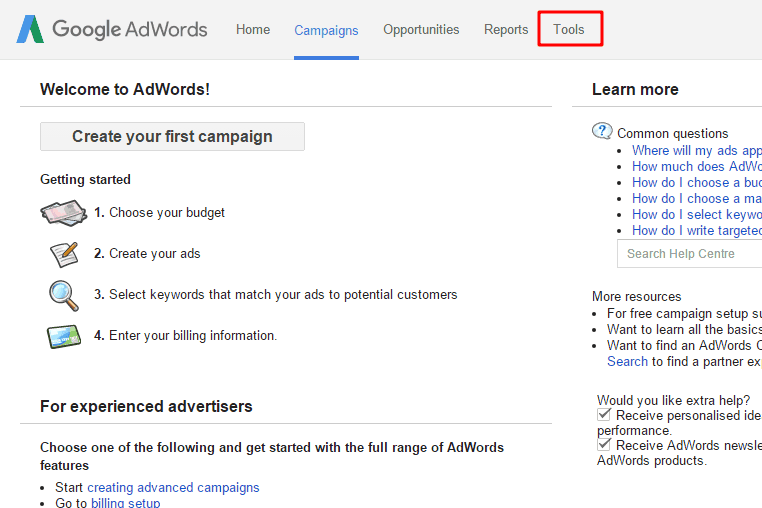The screenshot displays the interface of Google AdWords. At the top of the screen, a gray bar features a blue horizontal line and a green downward-sloping line resembling the letter "A." The text "Google AdWords" is rendered in black, followed by navigation options: "Home,” “Campaigns” (highlighted in blue with an underline), “Opportunities,” “Reports,” and “Tools” (enclosed in a red square).

The central section prominently welcomes users with the message "Welcome to AdWords, create your first campaign," followed by a "Getting Started" guide divided into four steps, each accompanied by illustrative icons. Step one, represented by a stack of papers, instructs users to choose their budget. Step two, depicted with a pen writing on paper, advises creating ads. Step three, explaining the selection of keywords to attract potential customers, includes textual guidance. Step four, concerning entering billing information, concludes the section.

For experienced advertisers, there is an invitation to access the complete range of AdWords features with blue hyperlinks labeled "create advanced campaigns" and "go to Billing Setup."

To the right, the screen provides links to "Frequently Asked Questions," "More Resources," and additional support information.